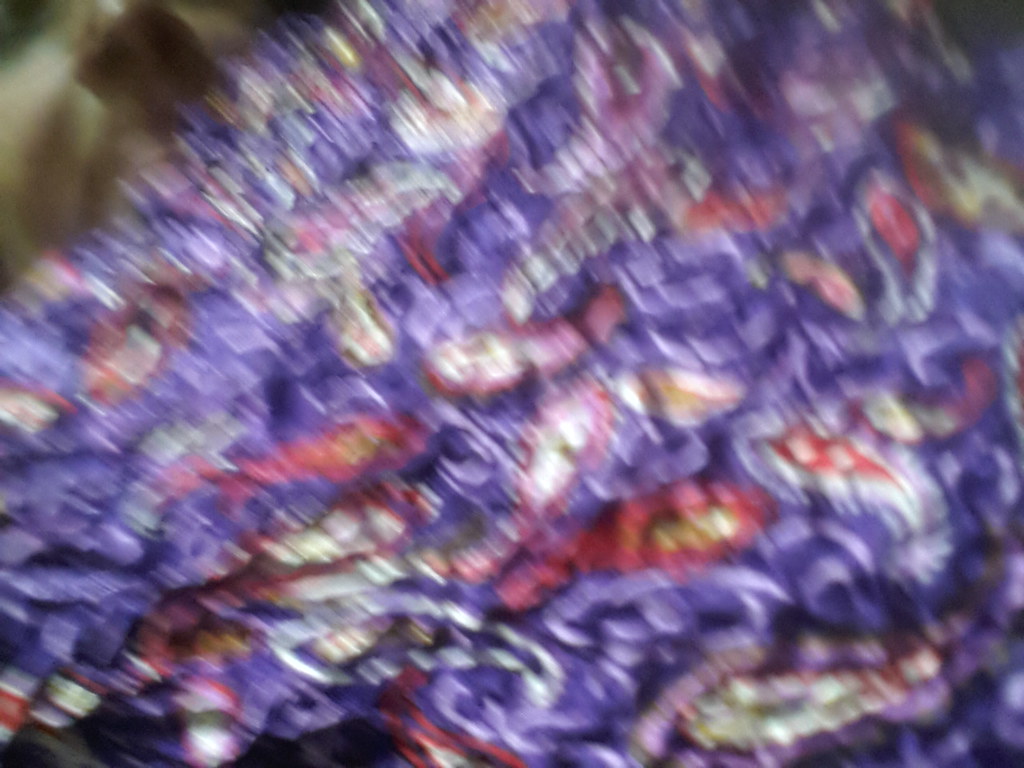This close-up photograph depicts a highly blurry and shaky image of a wrinkled, possibly silky piece of fabric, dominated by a purplish-dark blue color. The fabric features an intriguing pattern that appears to resemble small, brightly colored fish swimming in an ocean-like backdrop. These fish-like shapes vary in color, including red with yellow centers, white with orange centers, and pink with white centers, suggesting a consistent yet alternating pattern. The image quality makes it challenging to discern details, but additional colors such as gold, brown, and gray can be seen, particularly in splotches on the left side of the photo. The fabric itself exudes a shiny texture, adding to the impression that it could be a silky blanket or garment. Despite the lack of focus, the colorful and dynamic arrangement stands out against the purple background, contributing to the lively, aquatic-themed aesthetic.